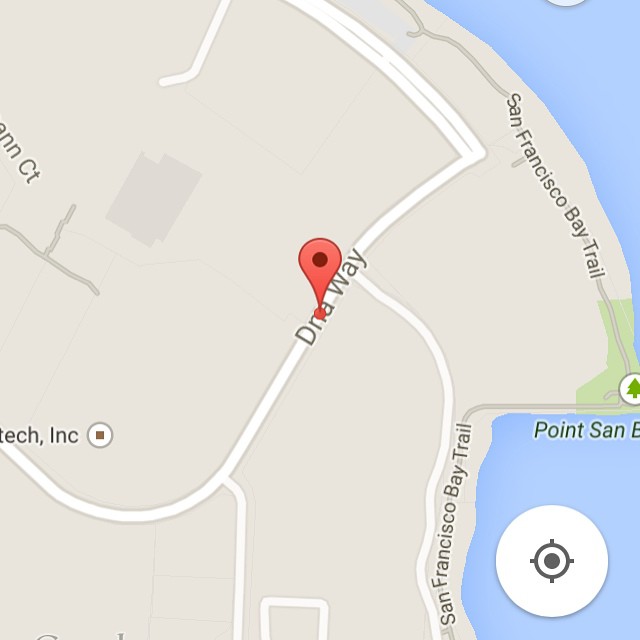A detailed portion of a map is depicted, prominently featuring a network of roads. The map covers almost the entire view with its light gray background and white road lines. In the upper right and lower right corners, patches of blue represent bodies of water. A medium gray line runs along the top of the map, labeled "San Francisco Bay Trail." The central roadway, labeled "DNA Way," cuts through the middle of the map. An unmarked white line branches off from "DNA Way." Additionally, there is a partially visible word at the end of this white line, though it is cut off and unreadable. The overall composition of the map indicates a focus on the infrastructural layout within this specific area.